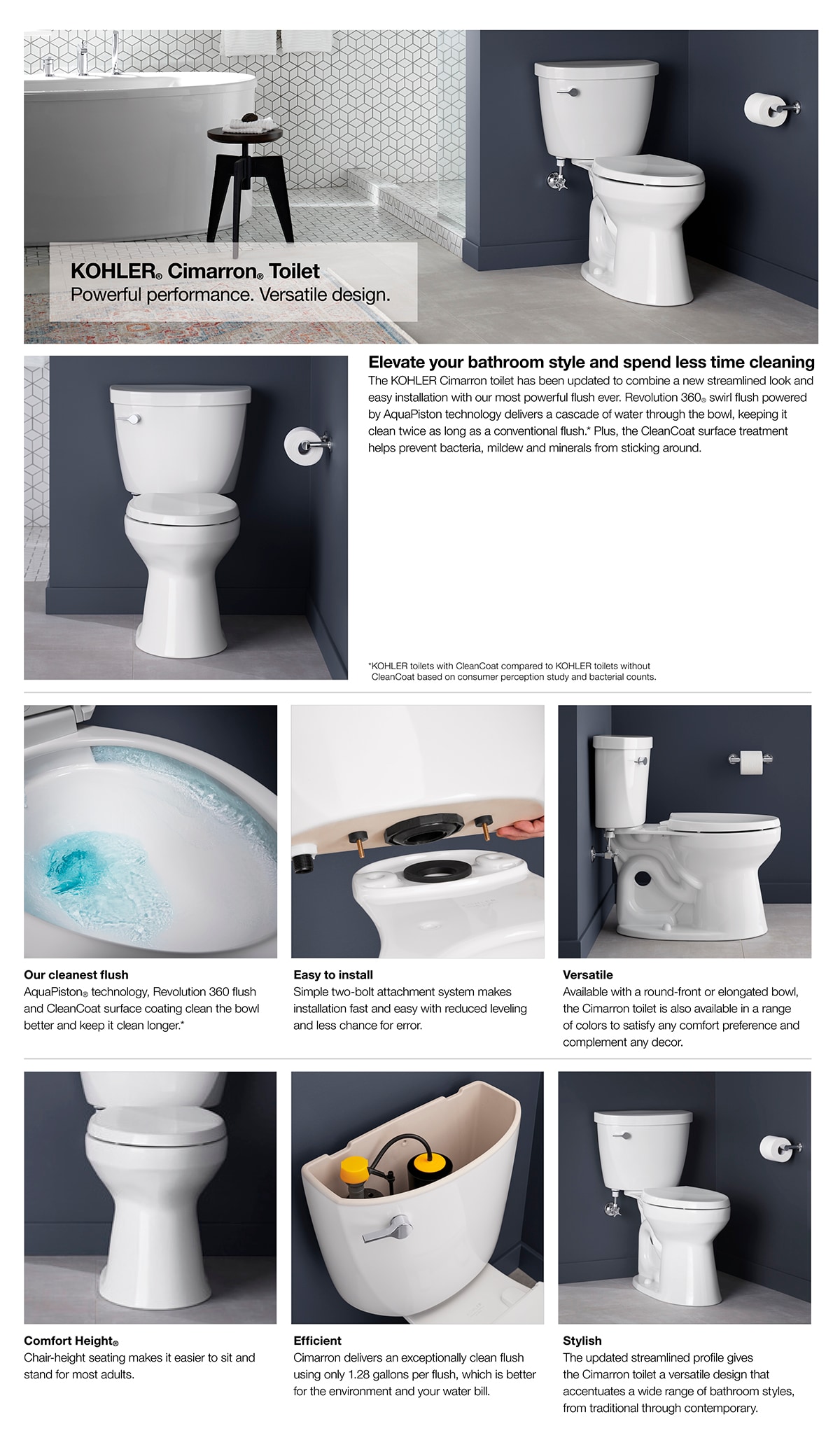This detailed image caption showcases a color advertisement for a Kohler toilet collection, specifically highlighting the Kohler Synmaroon Toilet. The ad features a series of eight photographs demonstrating the toilet's powerful performance and versatile design. Prominent in these staged pictures is a pristine, immaculately cleaned bathroom setting, with a striking deep blue wall behind the white toilet, enhancing its visual appeal. The bathroom also hosts a round jacuzzi-style bathtub, a shower, and line-styled wallpaper, contributing to a sophisticated ambiance. 

At the top, the ad proclaims: "Kohler Synmaroon Toilet — Powerful Performance, Versatile Design," emphasizing its stylish, easy-to-install construction, clean flush, comfortable height, and efficient water flow. Accompanying the main image, additional snapshots show the toilet from various angles, highlight features such as the efficient flush system, installation process, and overall versatility. The thorough design and performance advantages position this model as superior to competitors, all while promising to "elevate your bathroom style and spend less time cleaning."